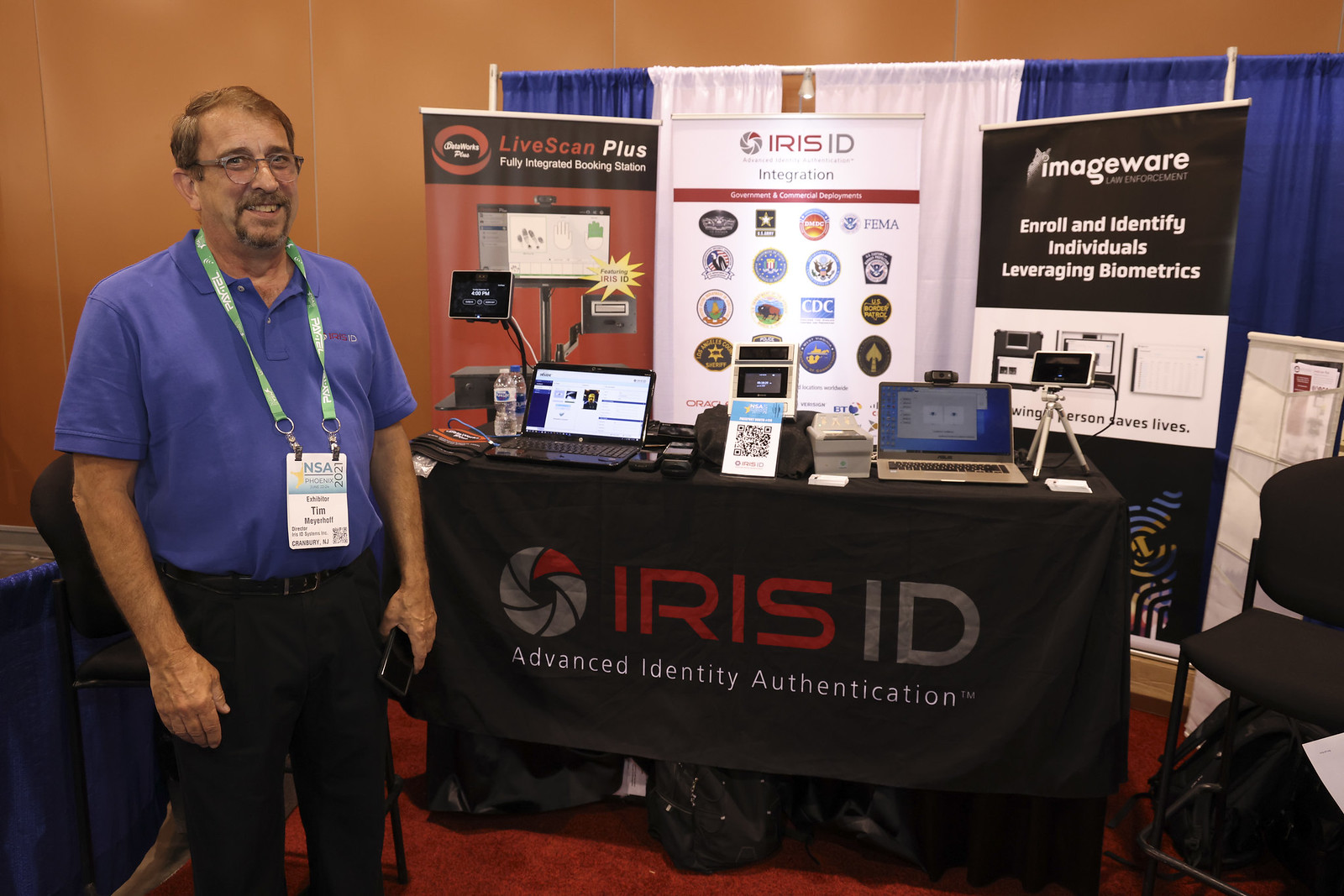The image features a man standing to the left of a table draped in a black tablecloth with the logo "Iris ID" in red and gray lettering, followed by "Advanced Identity Authentication" in white. The man, identified as Tim from his NSA 2021 ID badge hanging on a lanyard around his neck, is smiling and dressed in a blue button-down shirt paired with black pants and a black belt. He sports a goatee and stands in front of a conference stand with the same Iris ID logo. Behind him are multiple laptops and three vertical backdrop posters promoting related products and services. The first poster, in red and black, advertises the "LiveScan Plus Fully Integrated Booking Station." The second poster on a white background displays the Iris ID logo in red and gray. The third poster, in black and white, reads "ImageWare Enroll and Identify Individuals Leveraging Biometrics." The image was taken at the NSA convention, suggesting a focus on advanced biometric authentication technology.